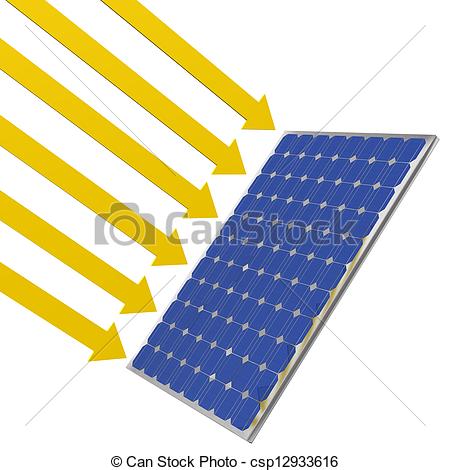The image features a blue solar panel with a silver frame, tilted diagonally on its side against a white background. The panel is made up of numerous small cells arranged in a grid. Dominating the left side of the image are six thick yellow arrows of varying lengths, all pointing towards the solar panel. These arrows originate from the top left corner of the image and gradually decrease in size as they approach the panel. The longest arrow starts from the very corner, converging on the blue surface of the panel. A watermark for "Can Stock" is prominently present, along with a small camera icon, indicating that this is a stock photo. Below the panel, the text "Copyright Can Stock Photo CSP 129 3 3 6 1 6" is visible.